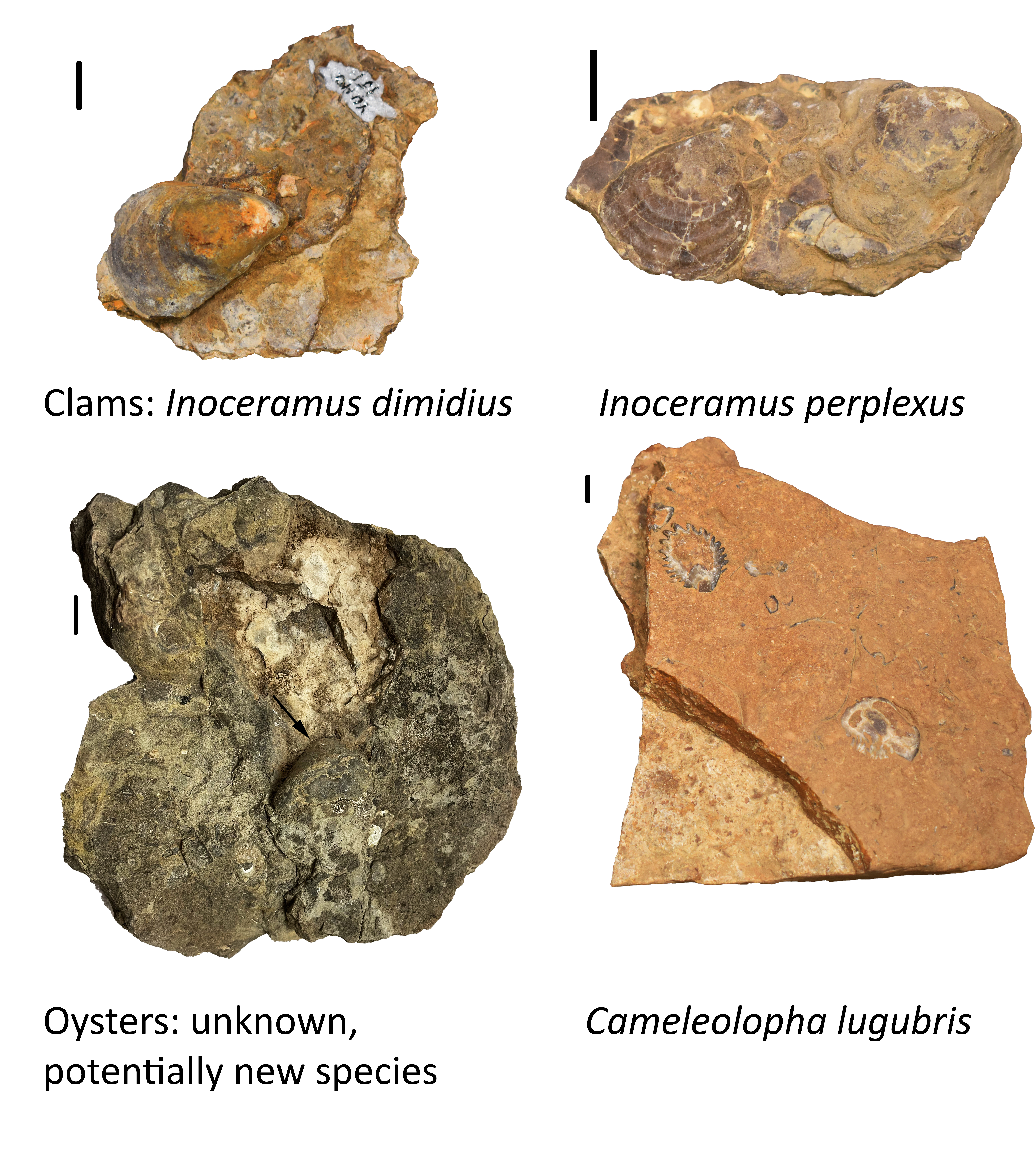This image showcases four distinct fossil-containing rocks, arranged in a 2x2 grid on a white background. Each rock is meticulously labeled with the species and scientific names. The top left rock, identified as "Clams: Inoceramus dimidius," is a mix of yellow, white, and brown. Adjacent to it, the top right rock labeled "Inoceramus perplexus," presents a golden-brown hue with black and gray spots. The bottom left rock, marked "Oysters: Unknown, potentially new species," is darker, predominantly grayish-brown with black and white areas. Lastly, the bottom right rock, almost square-shaped and an orangey-brown color reminiscent of terracotta, is labeled "Camellialofa lugubris." The rocks, appearing to contain smaller embedded fossils, suggest they are clam and oyster fossils rather than living organisms.